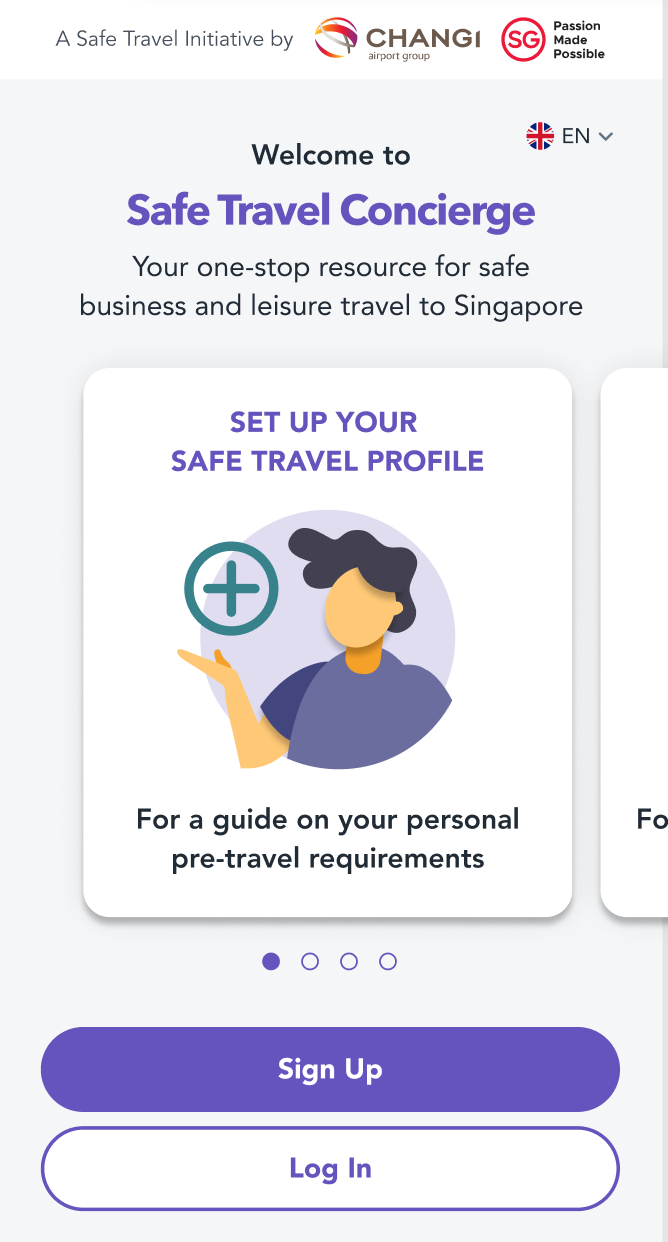The image showcases a webpage titled "A Safe Travel Initiative by Changi," with the text prominently displaying "SG" and the tagline "Passion Made Possible." It serves as an introduction to the "Safe Travel Concierge," which is described as a comprehensive resource for safe business and leisure travel to Singapore. The page features a circular icon with a British flag and the abbreviation "EN," indicating language options via a drop-down menu. Below, there are instructions to "Set Up Your Safe Travel Profile" and details on "your personal pre-travel requirements."

The visual elements include the outline of a faceless figure holding up a plus sign, symbolizing the creation of a travel profile. Other parts of the webpage are partially visible to the right, suggesting the need to scroll for more information. At the bottom, the page features navigation dots—one filled with a purple color and three empty—indicating the current step in a multi-step process. Two buttons are prominently displayed: a "Sign Up" button in a purplish hue and a "Log In" button in white.